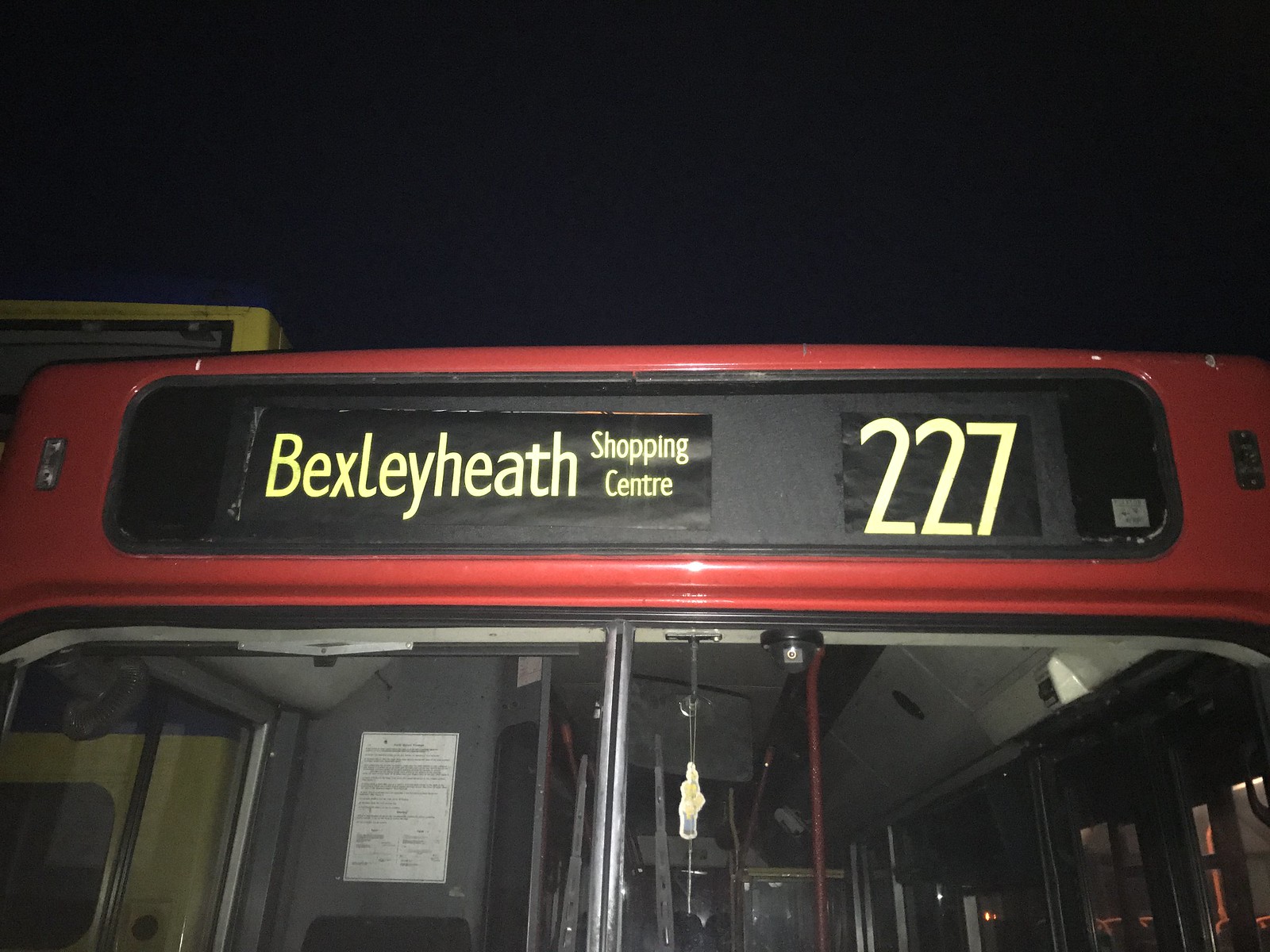This image captures a nighttime scene featuring the front upper portion of a red public transit bus parked outside under a pitch-black sky. The central focus is the bus's signage, which is bright yellow and prominently displays the destination "Bexley Heath Shopping Center" with the route number "227." The image reveals the bus's windshield and a glimpse of the interior, which is dimly lit and empty. A notable detail is an air freshener or an object resembling an image of Homer Simpson hanging inside the bus near the center of the window. The scene is devoid of people, contributing to the dark and quiet ambiance.